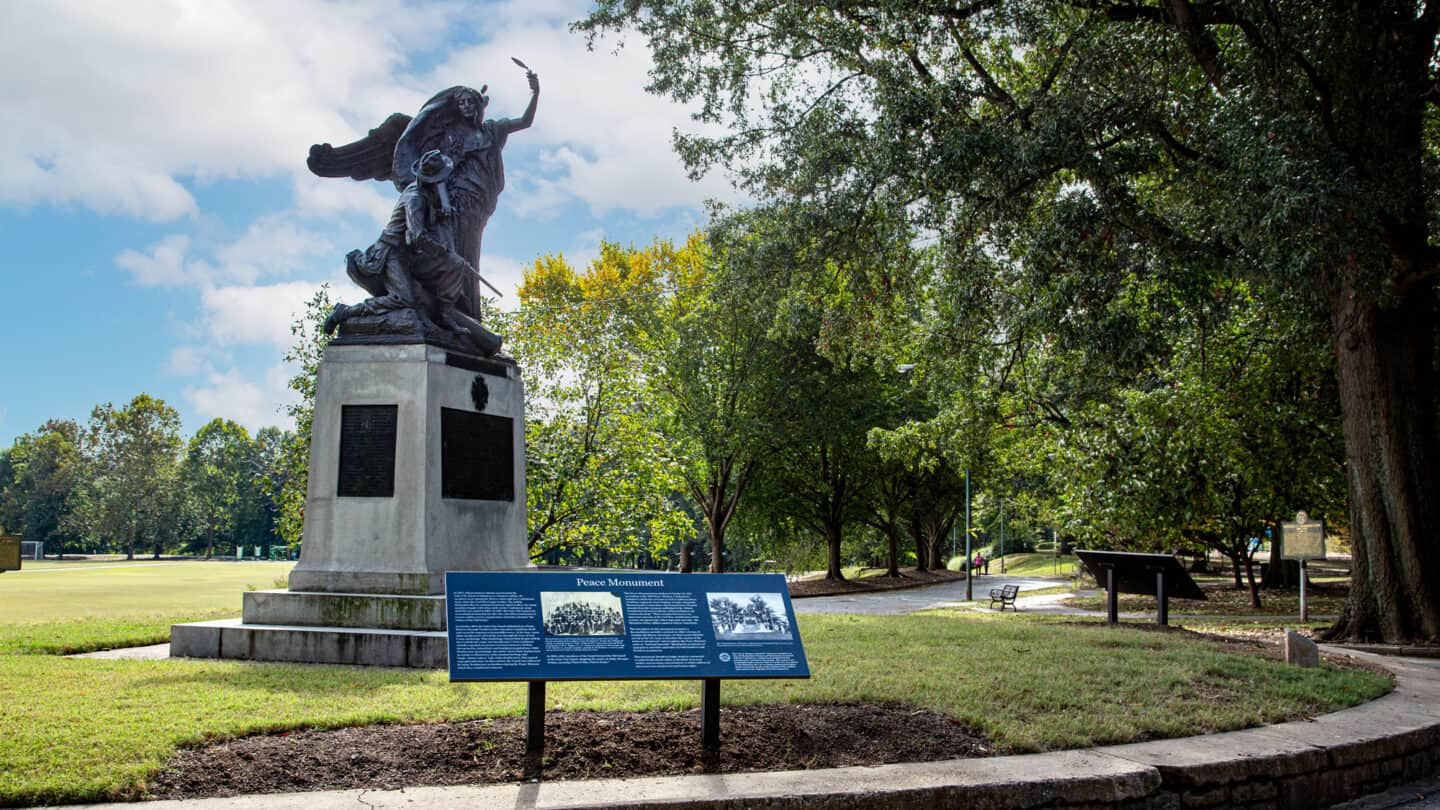In this image, we see the Peace Monument situated in a public park. The monument is approached by a semi-circular cement path and framed by a blue sign with a white border, supported by two black rectangular posts. The sign bears the name "Peace Monument" along with four columns of text and two small, indiscernible pictures. The monument itself is elevated on a flat mound of green grass and consists of several tiers: two steps form the base, supporting a large rectangular stone pedestal adorned with black plaques on its side and front. Atop the pedestal, a bronze-like statue depicts a poignant scene: an angelic figure, seemingly hovering or standing, with its arm raised as it faces a kneeling military man who holds a gun and wears a hat. The backdrop of the park features numerous trees, set against a partly sunny sky.